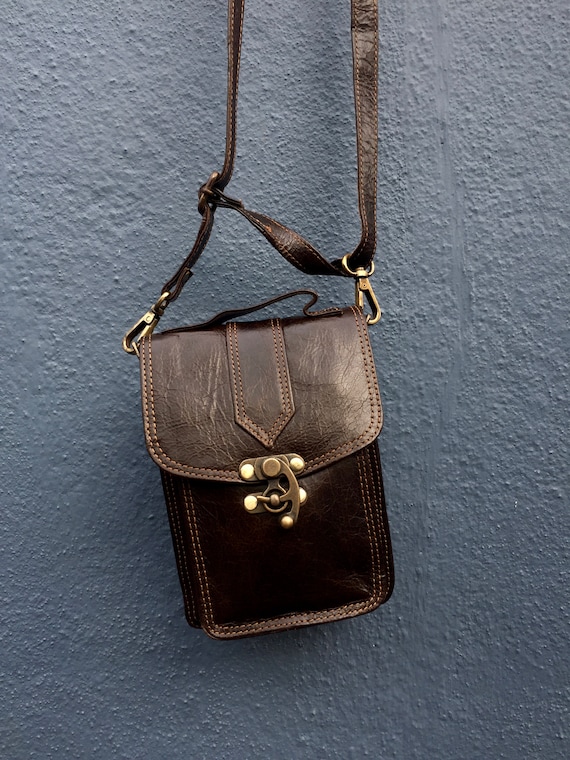The image depicts a dark brown leather handbag or purse, designed in a vertical rectangular shape, ideal for cross-body wear due to its long leather strap. The bag features intricate detailing such as heavy, double stitching around the edges, adding to its durability and aesthetics. It has a prominent clasp in the center to secure the flap, which is silver with five white buttons. The leather strap is attached to the bag with gold-colored metal connectors. The background is a light gray stucco wall with a rough, stippled texture, providing a neutral backdrop that highlights the rich brown color of the leather. The purse is hanging from an unseen hook, positioned centrally in the image.